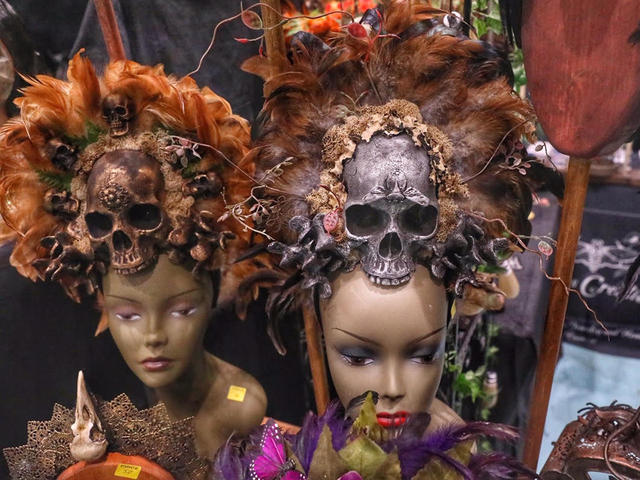In an ornate and busy scene set within a colorful shop, possibly an antique or secondhand store, two mannequin busts, each meticulously detailed, are on display. Both mannequins reveal only their shoulders and heads, adorned in lavish headdresses featuring prominent skull motifs. The tan mannequins, one representing an African American woman with red hair and a bronze skull atop her forehead, and the other a white woman with wild hair crowned by a silver skull, exude a strong sense of cultural ritual, possibly evoking themes of Halloween, Mardi Gras, or voodoo. The skulls, complemented by an array of burnt orange and tan feathers, small skulls, and various adornments including green, pink, purple, and pink butterfly decorations, make the picture feel exceedingly vibrant and detailed. The backdrop includes grey and blue hues with merchandise and elements like a wooden pole adding to the bustling ambiance. The mannequin on the right wears red lipstick, contrasting with the bare lips of the one on the left, enriching the layered, almost mystical atmosphere of the scene.